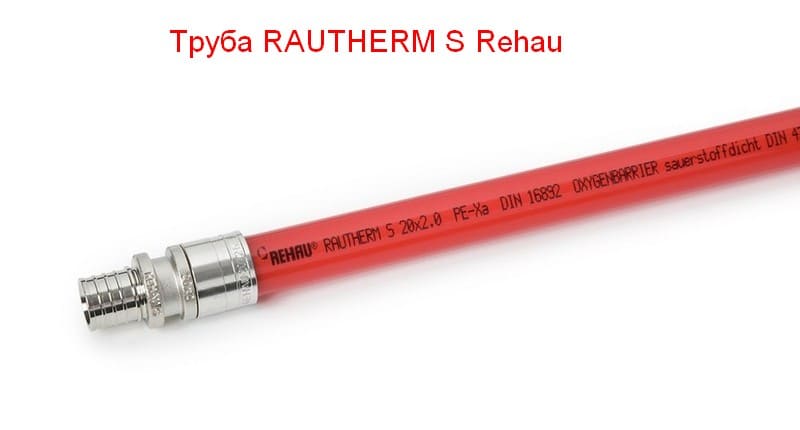This photograph features a bright red tube extending horizontally across a pristine white background. The tube, which resembles the shape of a pencil, is adorned with black text that reads: "Reri Rotherm S 20 by 2.0 PE-XA DIN 16892 Oxygen Barrier Sarsdorf Ditch DIN 47." This suggests it is designed to transport liquid or gas, likely as part of an advanced piping or cabling system. On the left end of the tube, there is a shiny, silver metal connector that appears cylindrical, resembling a wrench, which likely facilitates attachment to other equipment. At the top of the image, prominent red text states: "TPY6A Rotherm S REHAU," potentially identifying the model or brand of the tube and its components.